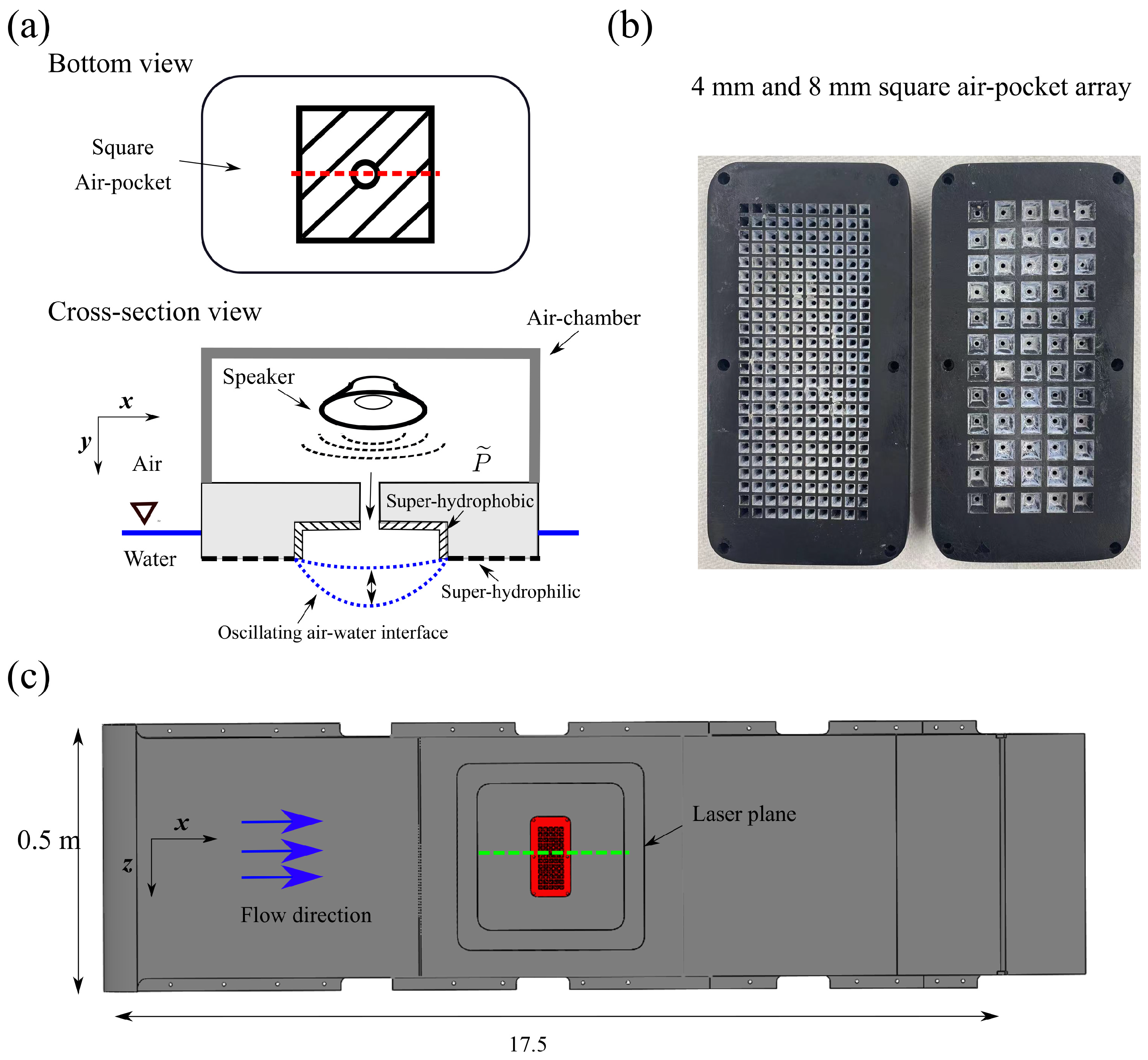This technical diagram, set against a white background, is divided into three labeled sections: A, B, and C, each illustrating different aspects of a detailed process. 

Section A, located at the top left, features both a bottom view and a cross-sectional view of a square air pocket. The bottom view includes text annotations and visual elements such as a rounded rectangle containing a striped square with a central circle and a segmented horizontal line. The cross-sectional view beneath it labels various components, including a speaker and distinct zones like air, water, superhydrophobic and superhydrophilic areas, and oscillating air-water interfaces.

Section B, centrally located, presents two photographs of similar black, potentially metallic objects. Text at the top of this section labels them as 4mm and 8mm square air pocket arrays. These vertical rectangular devices have grids of small squares, with the left object displaying smaller squares compared to the right.

Section C, situated at the bottom right, shows a gray rectangle denoting a flow direction and laser plane system. This section features three blue arrows indicating rightward flow, an X-axis pointing right, and a Z-axis pointing downward. Additionally, it includes measurements of 0.5 meters in height and 17.5 meters in length, as well as further detailed labeling within the rectangle, which contains a smaller square and a rectangle with a dotted green line.

The overall diagram provides a detailed and annotated technical overview that combines cross-sections, photographic comparisons, and schematic representations to convey complex information clearly.